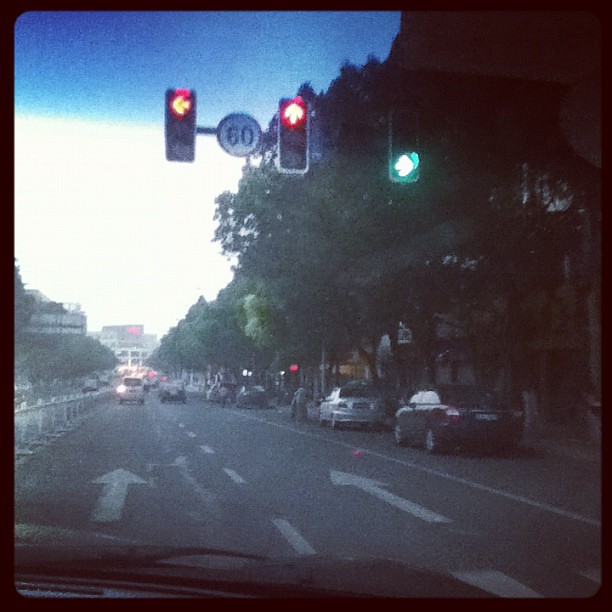The photo, taken from inside a car through the windshield, showcases a street scene with a traffic light. The image has a retro, grainy tone, reminiscent of a 2013 Instagram filter. At the intersection ahead, there are three streetlights with arrows: the left and middle arrows are red, indicating a left turn and going straight, respectively. The right arrow is green, signaling a right turn. Positioned among these lights is a circular speed limit sign with the number 60 in black. The road has two lanes with white forward-pointing arrows painted on it. To the right, there are trees, beige buildings, and parked cars, with one person visible exiting a vehicle. Other cars populate the road and are visible on the opposite side of the intersection, blending into the urban setting.